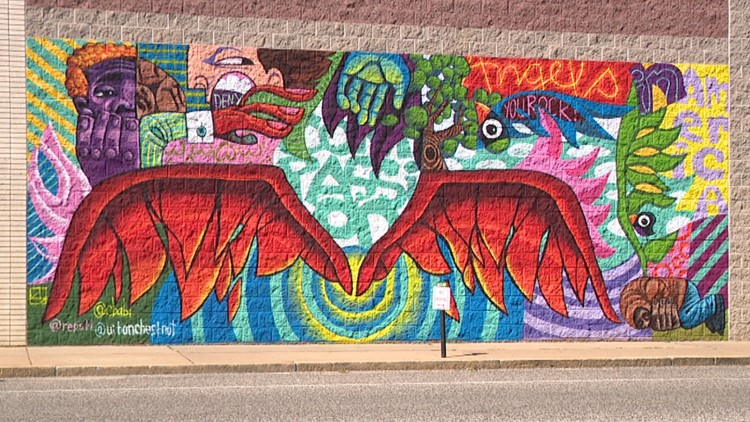This is a photograph of a vibrant mural painted on the side of a tan, brick building. The mural is created in a bold, cartoon-like style and features an array of bright, eye-catching colors. Dominating the artwork is a pair of radiant red wings emerging from a yellow Sun, which radiates yellow and blue circles. Above the wings, a tree is depicted, alongside several pairs of hands, including a prominent red pair extending from a green striped shirt. The mural also includes at least three human figures, one with a purplish face and orange hair and another with a peach-colored face and brown hair. The words "You rock" and "America" are prominently displayed, with "America" styled vertically with each letter stacked. There's also a green plant with a small bird perched on it and some at-symbols at the bottom left, hinting at the artist's identity. The scene includes a sidewalk in front of the mural and a street, with a no parking sign visible, adding to the urban context of the artwork.